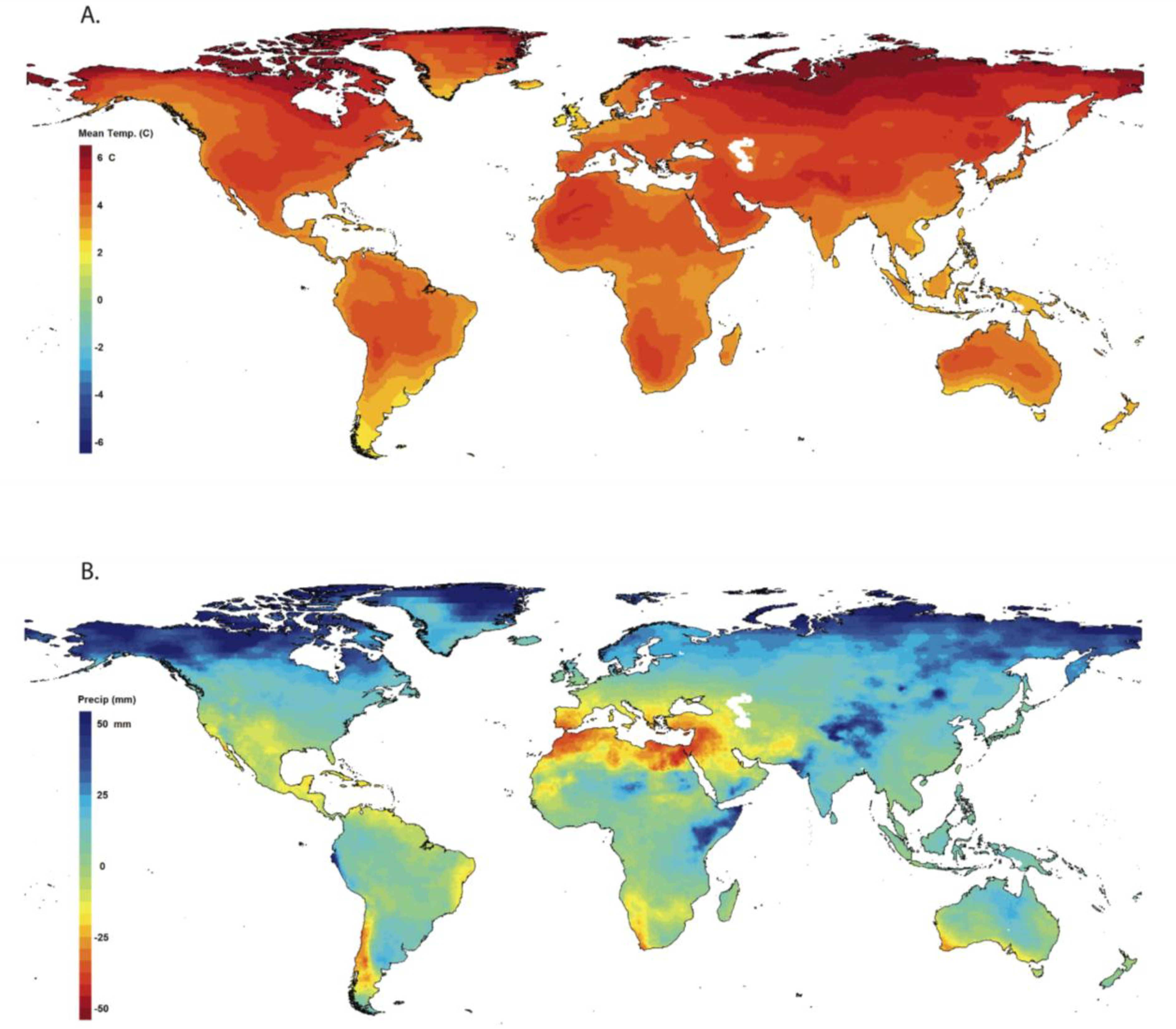This image presents two side-by-side flattened world maps with a color-coded legend on the left. The top map, labeled "A," displays mean temperatures in Celsius. Countries are depicted in various shades of red, orange, and yellow, with intense dark red and even black regions around some northern areas, indicating higher temperatures. Notably, the southern tip of South America shows a yellow hue. The bottom map, labeled "B," represents precipitation levels and is predominantly blue, varying from dark to light shades, with occasional specks of yellow and red, particularly around Africa and Europe, suggesting varying precipitation intensities. The legend on the left ranges from dark blue to bright red, illustrating the different temperature and precipitation levels across the maps.